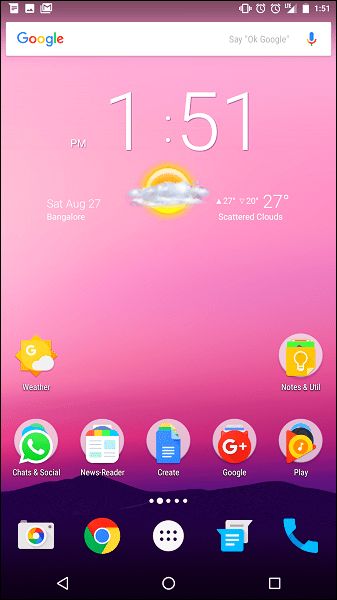The screenshot features a smartphone's home screen with a vibrant, gradient background. The top inch of the screen is a dark purple, transitioning to light pink about halfway down. From there, the color shifts to a darker purple and finally to a very dark blue at the bottom two inches, resembling a mountain range silhouette.

In the top left corner of the screen is a small white square, next to which are icons for a photo gallery and Gmail. On the top right, the time reads "1:51 PM," accompanied by a full battery icon, an internet signal icon at three-quarters strength, two alarm indicators, and a vibrate mode symbol.

Below, a white search bar with a Google logo on the left and a microphone icon for Google Voice on the right is displayed. The text inside the search bar prompts, "Say OK Google."

Under the search bar is a large white digital clock displaying "1:51 PM." To its left is a small "PM," and beneath it, a weather widget with a sun partially obscured by a cloud, reading "Saturday, Aug 27, Bangalore." It indicates a temperature range from a high of 27 degrees to a low of 20 degrees, currently showing 27 degrees Celsius with "scattered showers" specified.

As the color begins to darken, icons for weather and notes/utilities appear on the left and right side, respectively. A row of five icons follows: "chat and social," "news reader," "create," "Google," and "play."

At the bottom section, five white circles are centered, representing different functions. The interface is rounded off with five primary icons along the bottom: camera, Chrome browser, settings, messaging, and telephone. Lastly, the bottom center features a white circle home button, flanked by a white square for recent apps on the right, and a white triangle pointing to the left, symbolizing the back button.